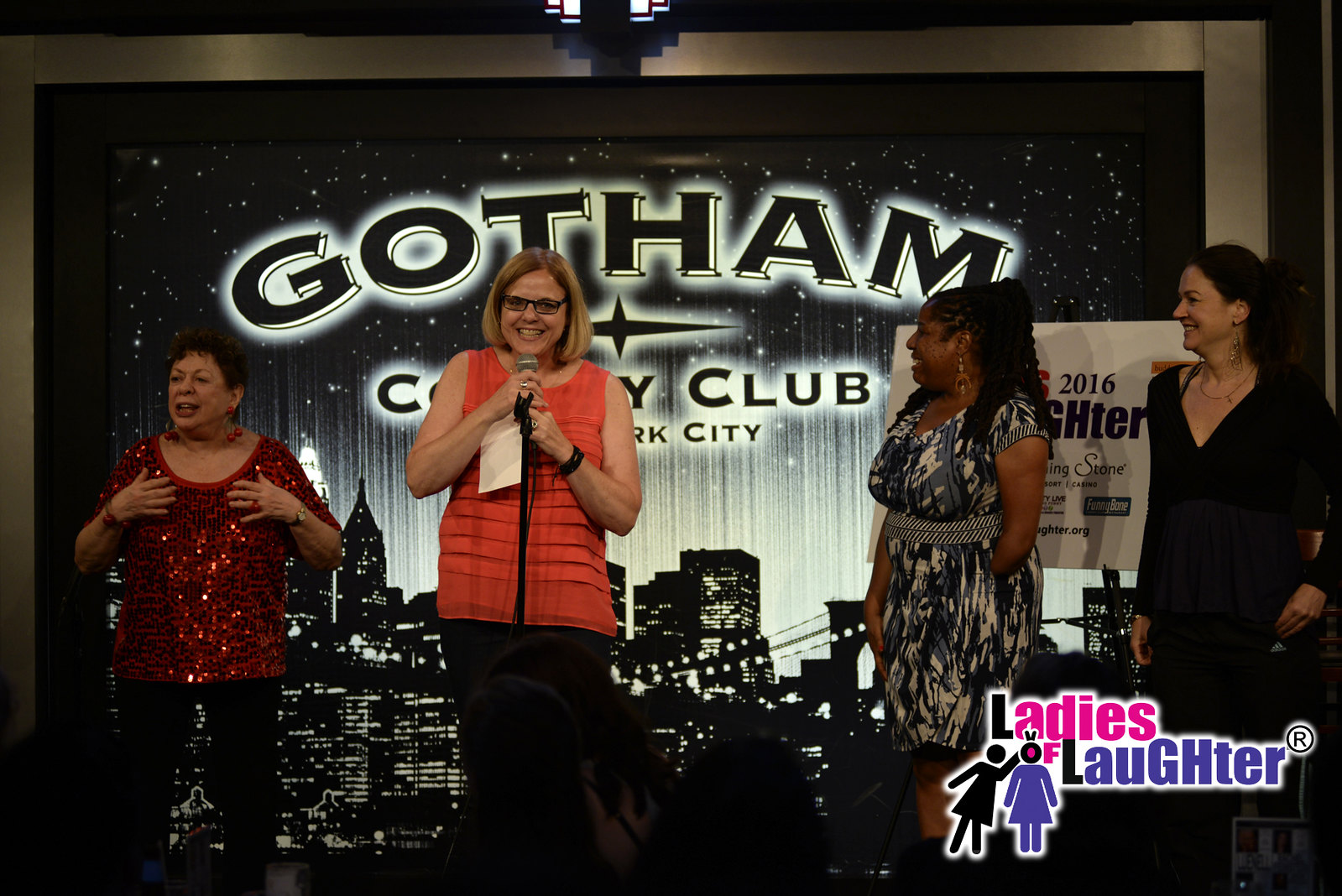In this vibrant photo captured at the renowned Gotham Comedy Club in New York City, four middle-aged comedians grace the stage, each engrossed in their unique act. Against the backdrop of a black and white New York City skyline adorned with twinkling stars, the club's name, "Gotham Comedy Club," is prominently displayed. Bright stage lights illuminate the scene, while a partially visible banner touts the year 2016 and phrases like "fighter," "stone," and "funny bone."

At the far left stands a woman in a red sequined top with black pants, her short black hair complemented by red cherry earrings and a wristwatch. She's animated, gesturing energetically towards the audience. Next to her, another woman with neck-length blonde hair and black-rimmed glasses holds a microphone fixed on a stand. Dressed in a sleeveless orange top and black pants, she exudes confidence as she engages the crowd with a wide smile. 

Beside her, a curvy woman with long curly black hair chuckles; her dress features a striking splatter pattern of blue, black, and white. She looks towards the audience, where interaction is lighting up the room. The final comedian, on the far right, is decked out in a sophisticated black ensemble with a deep neckline, large earrings, and a visible pendant. Her laughter matches the engaging atmosphere, directed at the audience participation.

The image is subtly branded with a watermark in the lower right corner, featuring the "Ladies of Laughter" logo, a testament to the comedic talent present in this lively portrait.